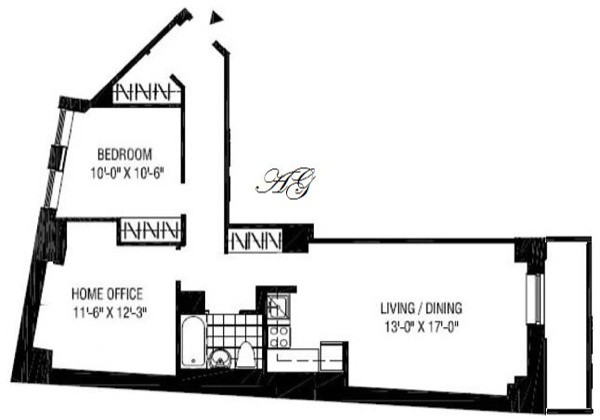The black-and-white floor plan showcases an L-shaped layout, meticulously drawn with precise, straight lines, suggesting it was either printed or hand-drawn with a black marker and ruler. On the left side, there is a 10x10 feet bedroom labeled "Bedroom." Adjacent to this room at the bottom edge, a home office measuring 11'6" by 12'3" is depicted, featuring a closet in its top-right corner. Moving right, a bathroom with a tiled floor design is positioned next to the bedroom. Although the bathroom dimensions are not specified, it includes a bathtub on the left, a sink in the center, and a toilet in the bottom right, with the door situated directly ahead.

Continuing to the right down the hallway, there is a spacious, irregularly shaped living and dining area, narrowing on the left and expanding on the right, labeled "Living/Dining" with dimensions of 13x17 feet. Furniture lines in the lower left corner of this room suggest the placement of a sofa and a chair. Opposite the bathroom, at the top of the hallway, lies the front door, providing an exit from the floor plan.